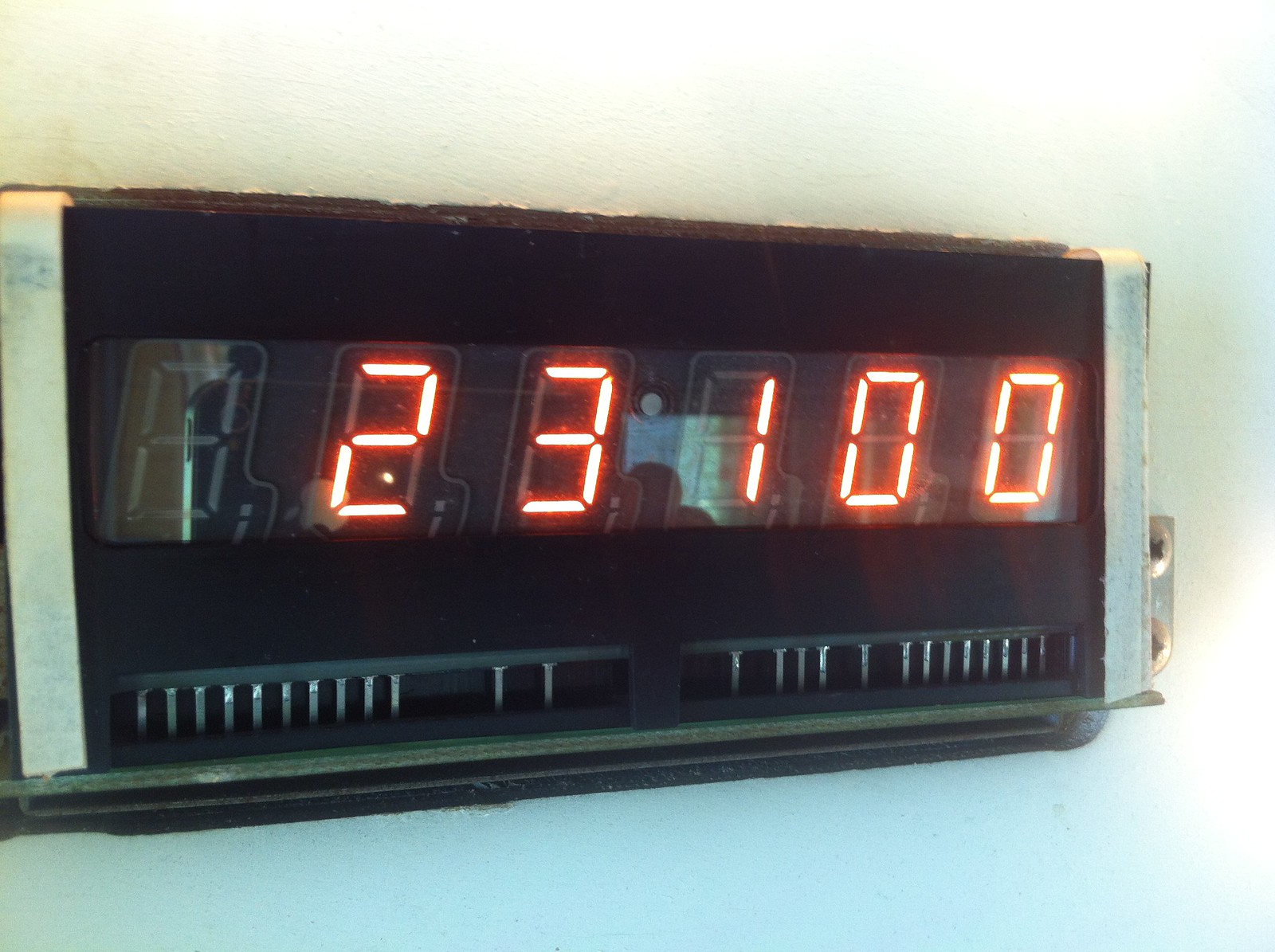In the image, a predominantly white background serves as a stark contrast to the central focus—a clock with a predominantly black face. Positioned centrally, the clock face features subtle reflections, adding a touch of realism and depth to the scene. Flanking the clock on both the left and right are light bars, which help illuminate the face and emphasize its sleek design. At the bottom of the clock face, a series of dashes are visible, possibly indicating minute markers, enhancing the clock's functionality and aesthetic.